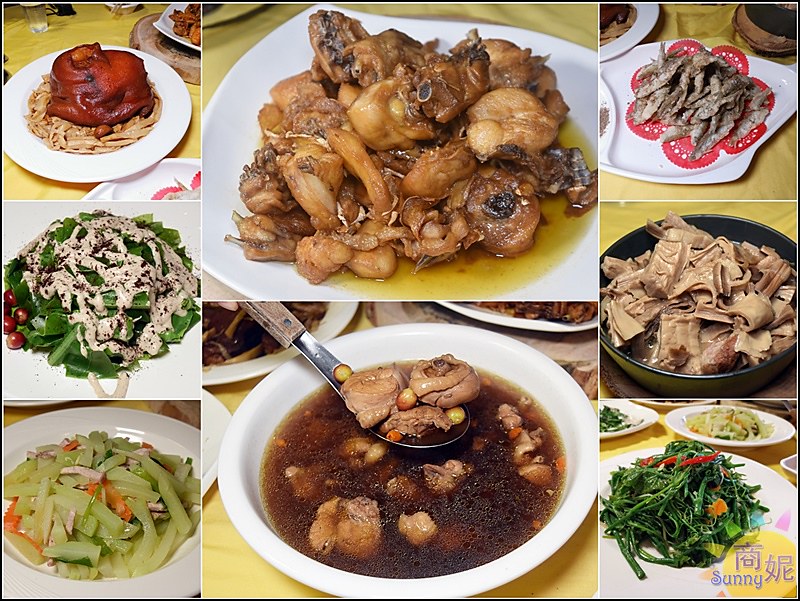The image is a collage of eight distinct photographs showcasing a variety of Asian entrees, each presented on unique dishes and platters. The layout features three smaller images on both the left and right columns, with two larger images in the center. The dishes appear to include elements such as greens with dressing, a variety of vegetables, and noodles topped with meat. In the center-left, there's a photograph of a meat dish with bones, served in a sauce on a white plate, and below it, a dark-brothed soup with chunks of meat, perhaps containing mushrooms. On the top right, there's a plate of whole tiny fish on a white dish decorated with a red doily. Below this, some cuts of possibly internal organ meats are presented in a black bowl, and underneath, a plate featuring green leafy vegetables. The collage captures the essence of Asian cuisine, likely Japanese as suggested by the oriental symbols in the lower right corner next to the English word "SUNNY".